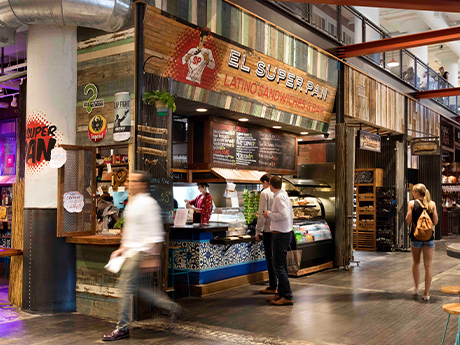The image is a daytime photograph taken indoors at a mall or food court, capturing a bustling corner of a shop. Central to the scene is a blurry man, light-skinned and dressed in a long-sleeved white shirt and gray dress slacks, walking from left to right. To his left stands a small eatery called "El Superpan," recognized by its distinct signage featuring an image of a man opening a shirt with the letters "SP." Above the store in bold white text against a brown background it says "El Superpan." Below this, red lettering reads "Latino Sandwiches and Bar." The store's front also displays handwritten menu items on blackboard-style panels. Behind the counter, a woman is busy preparing food for customers. Standing at the counter are two men in white long-sleeved shirts, blue pants, and brown boots. Near the right edge of the frame, walking away, is a woman with long brown hair, wearing blue jean shorts and a black tank top, carrying a brown bag. Above, the second level of the mall is visible, featuring a plexiglass barrier with a black metal frame and several people walking. The architectural details include red metal beams running horizontally across the upper right portion of the image. The floor is a brown linoleum, contributing to the overall warm, inviting atmosphere of the setting.